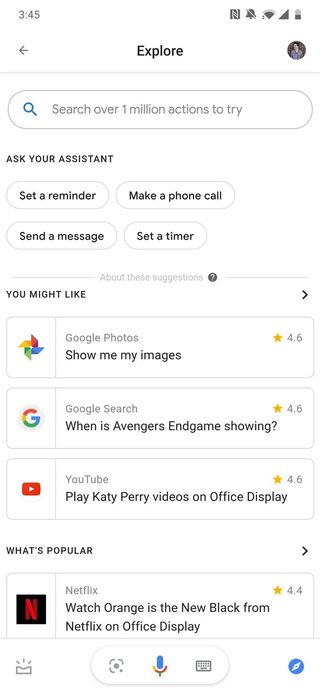The image shows a smartphone with a predominantly white background and black font. At the top, the current time and phone information are displayed. The screen is on a section titled "Explore," with a back arrow on the left side and an account icon on the right.

Below the "Explore" title, there is a search box with the placeholder text, "Search over 1 million actions to try." Underneath, in bold black font, the text "Ask your Assistant" appears, along with suggestions such as "Set a reminder," "Make a phone call," "Send a message," and "Set a timer." These suggestions are likely for Google Assistant, indicated by the recognizable Google colors.

A light gray font separates this top section from the lower section, which begins with the text "About these suggestions." Below, there are recommended actions categorized under "You might like." Another section titled "What's popular" provides additional suggestions, although the lower part of this section is partially cut off due to the screen's bottom edge.

At the very bottom, there are various interactive buttons, including options for speaking into the microphone, taking a picture, typing a suggestion, and other functionalities located on the left and right sides.